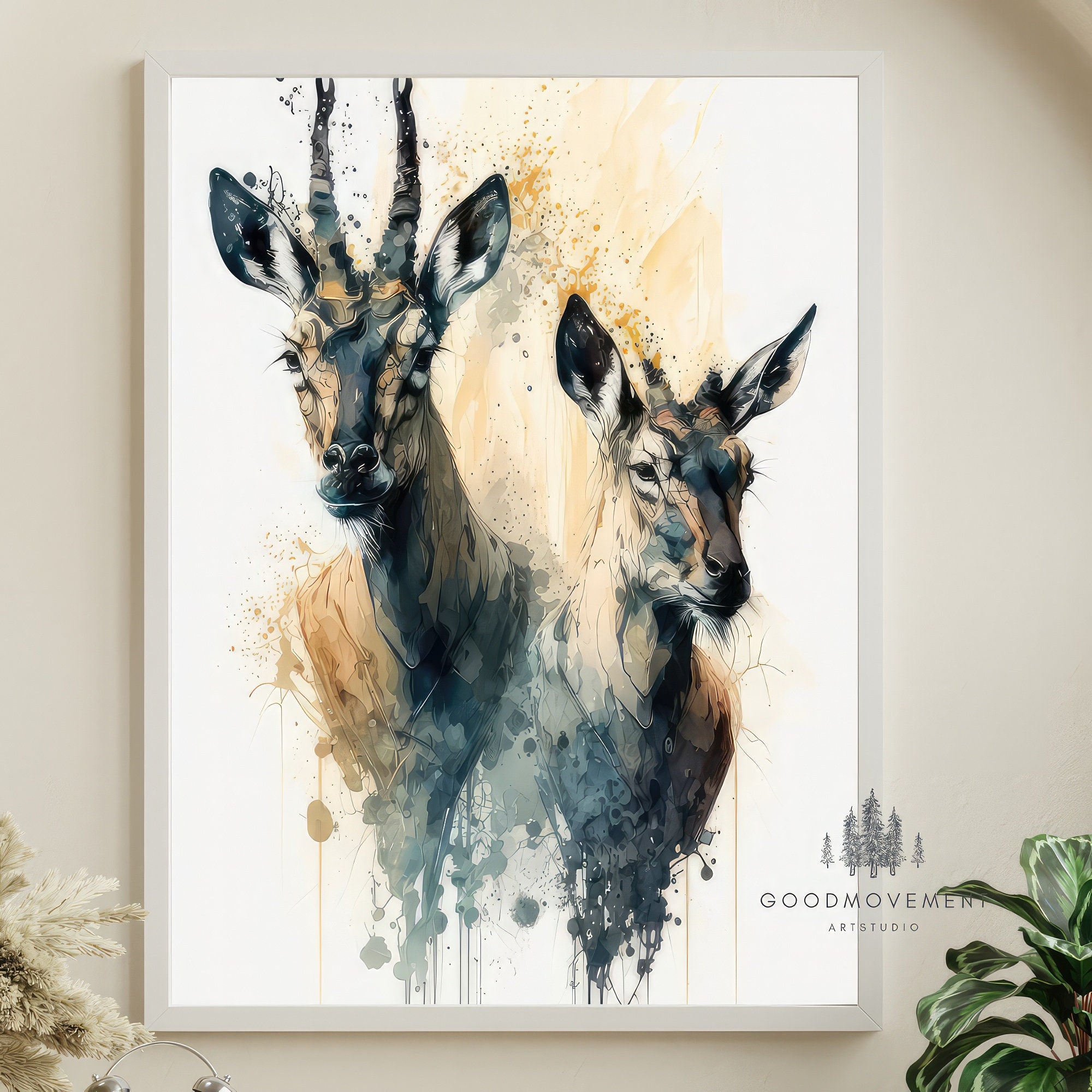A large framed canvas painting hangs on a white wall, with two deer-like animals depicted in an abstract style at its center. The animals, possibly caribou, have distinct features; one has long, vertical horns with a slight curve, while the other is shorter with smaller antlers. Both figures display a gray coat with black and white trim around their ears and are shaded with gray dots and an abstract finish. The background behind the animals features hues of brown, yellow, and gray, enhancing the abstract nature of the piece. Positioned at the bottom of the frame are two plants, one resembling a white, possibly artificial, evergreen plant, and the other with large, floppy green leaves. In the lower right corner of the canvas, a stamp with black silhouettes of evergreen trees stands out, accompanied by the words "Good Movement Art Studio."